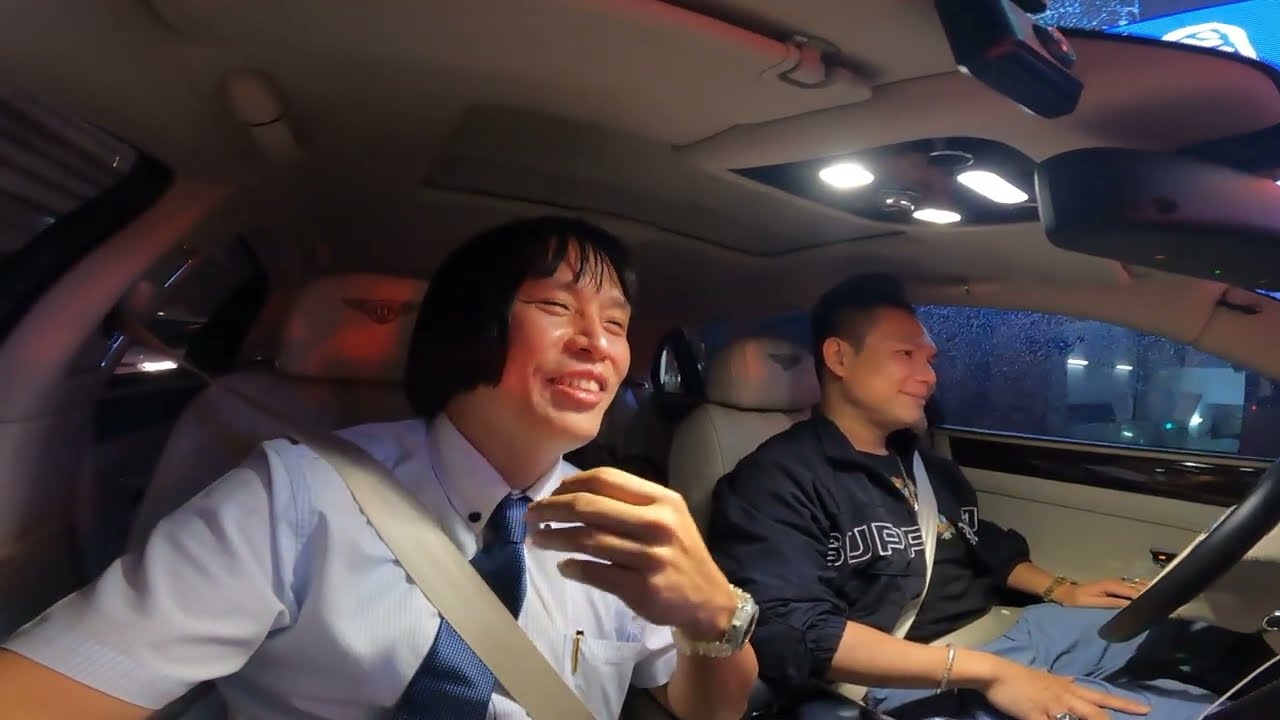This detailed, photorealistic image captures the interior of a car at night. The light tan interior, including the roof and seats, is softly illuminated by three overhead lights, casting a warm glow on the two Asian men seated in the front. The passenger, who has short black hair, is smiling broadly. He is wearing a light blue collared shirt paired with a blue tie, and a white watch on his wrist which he has raised up in front of his chest. He is capturing the moment with a selfie, a gesture highlighting the cheerful atmosphere. The driver, also smiling, has short black hair and is clad in a navy blue jacket with white lettering, with the sleeves rolled up, and blue pants. He sits comfortably with both hands rested on his legs, the black steering wheel visible in front of him. The darkness outside hints at nighttime, with subtle hints of exterior lights from a nearby building peeking through the windows, enhancing the cozy, intimate feel of the snapshot.